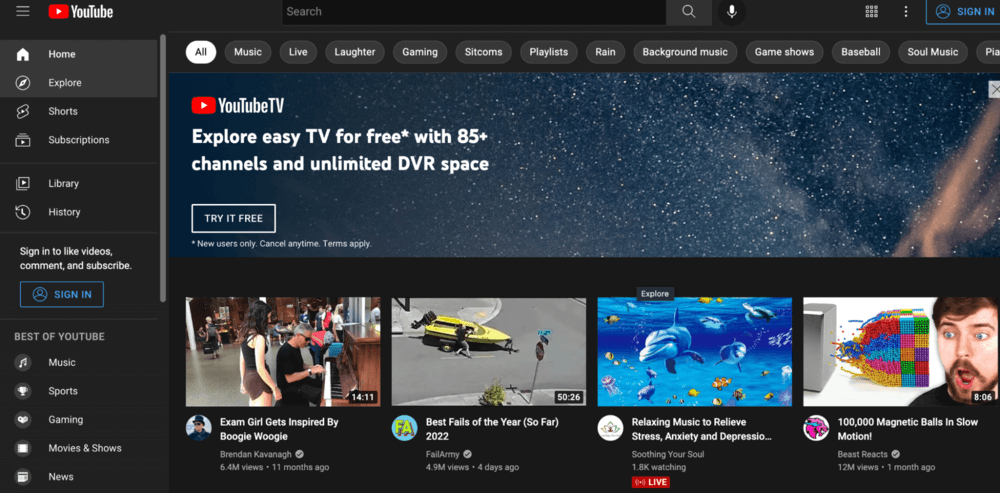This screenshot captures the homepage of YouTube as seen by a user who is not signed in, showcasing a variety of default recommendations and categories. Along the left sidebar, standard navigation options are visible, including Home, Explore, Shorts, Subscriptions, Library, and History. A prominent blue "Sign In" button invites users to sign in for personalized features such as liking videos, commenting, and subscribing.

At the top of the page, a horizontal menu offers quick access to popular YouTube categories: Music, Sports, Gaming, Movies, Shows, and News. The top of the screen features thematic tags like All, Music, Live, Laughter, Gaming, Sitcoms, Playlists, Rain, Background Music, Game Shows, and Baseball, allowing easy navigation through specific content types.

Additionally, there is a highlighted ad for YouTube TV, promoting a free trial with benefits such as access to 85+ channels and unlimited DVR space, stipulating availability for new users only with cancellation at any time under certain terms.

Displayed below the navigation options, four video thumbnails appear as suggested content:
1. "Exam Girl Gets Inspired by Boogie-Woogie" by Brendan Kavanaugh.
2. "Best Fails of the Year So Far 2022" by FailArmy.
3. "Relaxing Music to Relieve Stress, Anxiety, and Depression" by Soothing Your Soul.
4. "100,000 Magnetic Balls in Slow Motion" by Beast Reacts, a channel associated with Mr. Beast.

This snapshot provides a glimpse into YouTube's user interface and content offerings to an unsigned guest user.